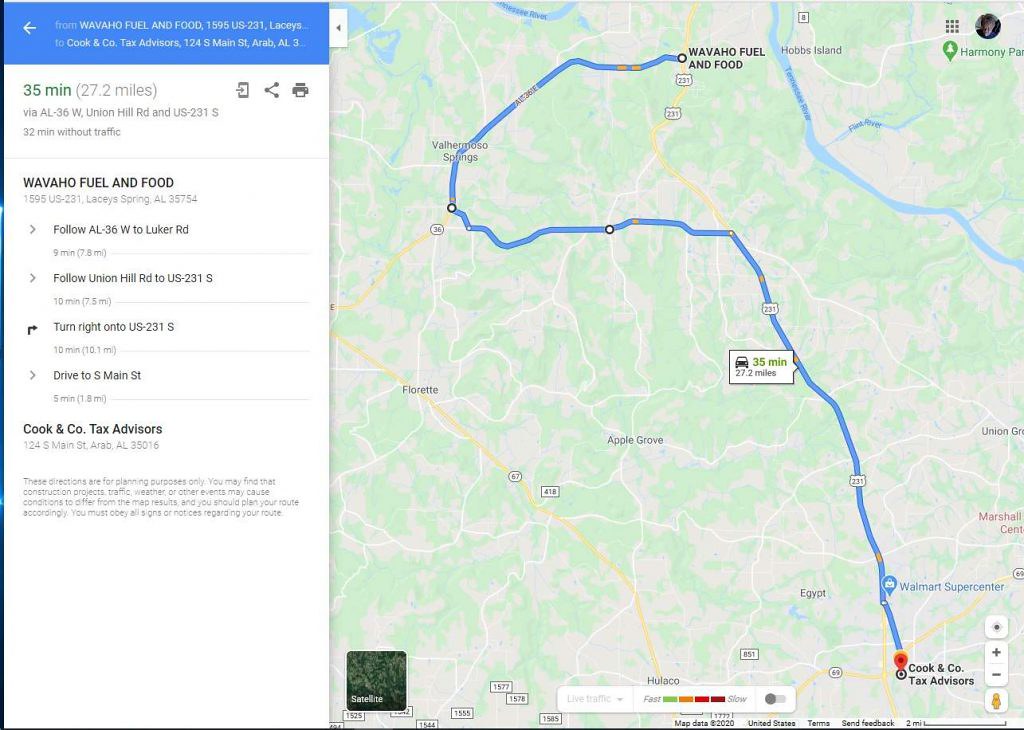This image showcases a detailed screenshot of driving directions from Wavahoe Fuel and Food to Cook and County Tax Advisors using Google Maps. The center of the image is dominated by the web page of Google Maps, displaying a color map with a dark blue route meandering 27.2 miles from the starting point at Wavahoe Fuel and Food, located on US 231, to the destination at Cook and County Tax Advisors. The travel time is estimated to be 35 minutes primarily via Alabama 36 West. The left side of the image features a column listing step-by-step driving directions. The map, set in the default map view, is predominantly green and tan, with a noticeable light blue river traversing it. Notably, the route passes by landmarks like a Walmart Supercenter shortly before reaching the final destination. Additionally, there are icons on the right for the user's login photo and functionality to adjust the map zoom level. The lower left corner shows an option to switch to satellite view, although the map view is currently selected.